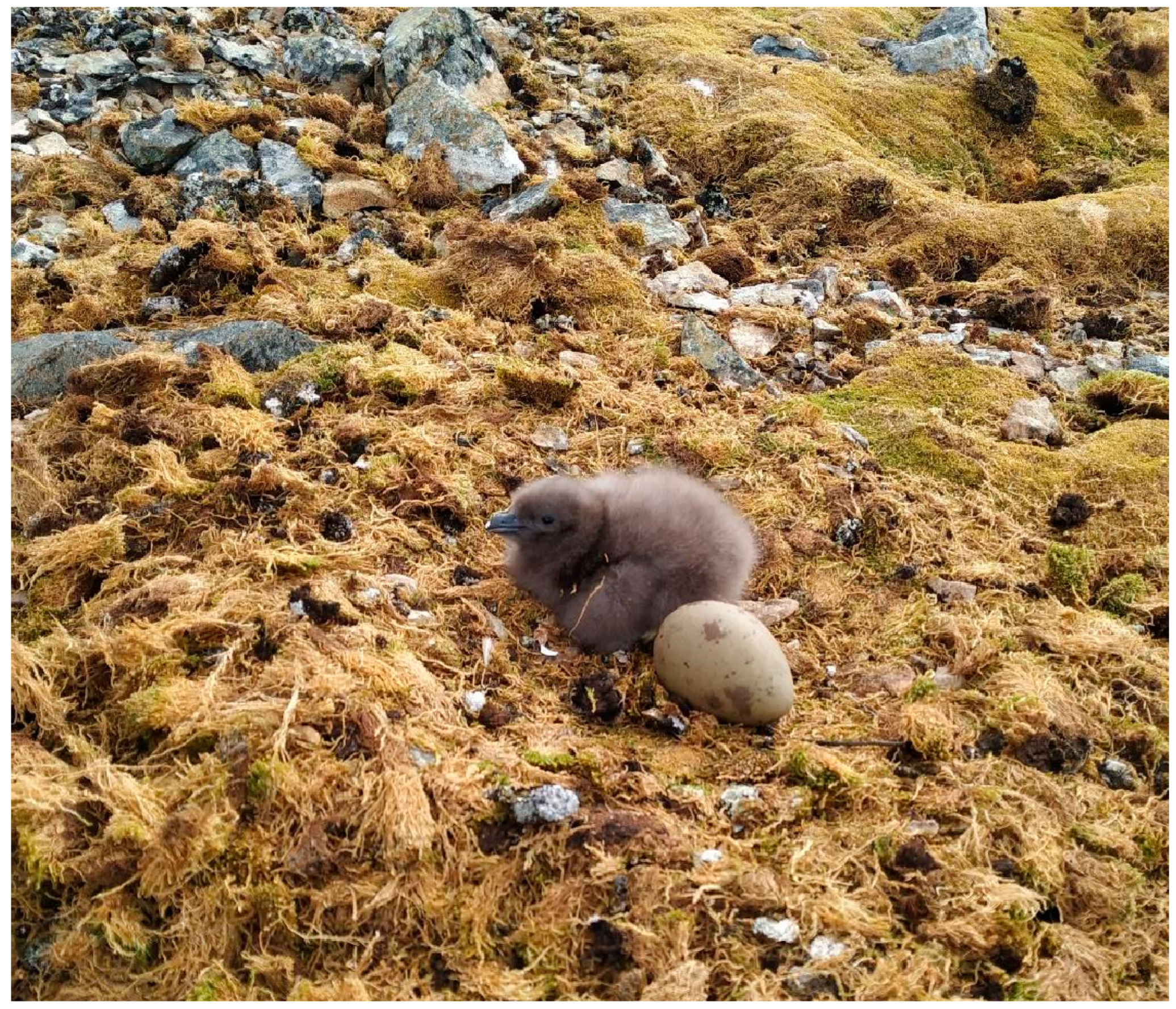In this color photograph taken outdoors during the day, a newly hatched Skua seabird chick is prominently featured standing on a hillside composed of gravel, small clumps of earth, and assorted gray and cobalt-colored stones. The environment is a natural landscape with rough hills and divots, transitioning from large stones to yellow grassy ground as the scene moves to the foreground. The fluffy, brownish-tan chick, with its black beak and small wings, stands in profile facing left, next to a large, oval-shaped egg that is light brown with dark brown spots. The egg is positioned slightly to the right and below the chick. The image captures the realistic, natural setting of this Antarctic bird in a square format photograph, emphasizing the intimate connection between the newly hatched chick and its earthy surroundings.